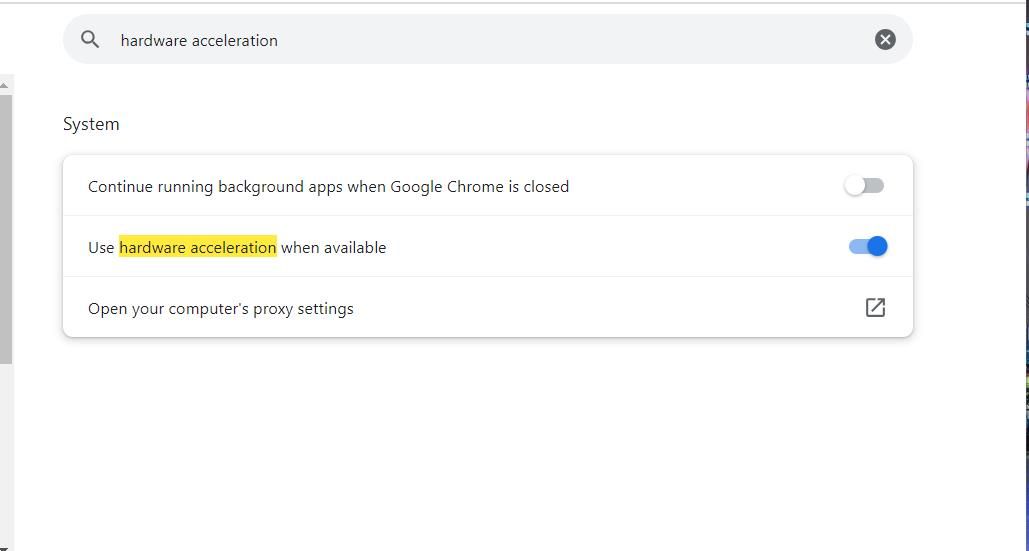The image depicts a straightforward interface set against a white background, featuring various search boxes and text in black or gray hues. At the very top, there is a gray search bar containing the text "hardware acceleration" with a small 'X' on the right end to clear the search. Below this search bar, there is a section labeled "System."

Within the "System" section, there are three adjustable settings:

1. "Continue running background apps when Google Chrome is closed," which is toggled off.
2. "Use hardware acceleration when available," with the phrase "hardware acceleration" highlighted in yellow to indicate relevance to the search query. This option is toggled on, evidenced by the blue switch.
3. "Open your computer's proxy settings," accompanied by a button on the far right for access.

On the left side of the page, a vertical scroll bar is visible, suggesting that more content might be accessible through scrolling. The focal point of the image is the highlighted "hardware acceleration" setting within the system menu, currently enabled as indicated by the blue toggle switch.